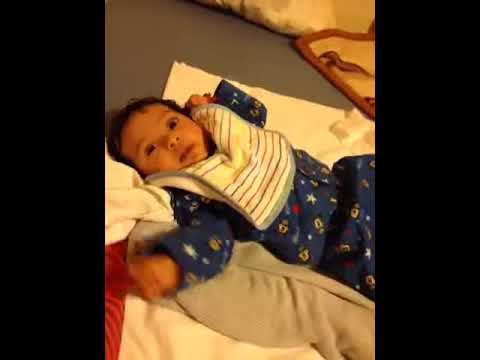The photograph is a color image in portrait orientation, with black borders on the left and right, making it taller than it is wide. The center of the image features a slightly blurry view of a young toddler with dark hair and dark skin, lying on a gray carpeted floor. The child, lying diagonally from the upper left to the lower right, looks upward to the upper left. They wear a dark blue long-sleeved onesie adorned with patterns of stars and horseshoes, and a large white bib with horizontal blue and red stripes, edged in gray. Surrounding the child are a white blanket and a fluffier gray blanket, with the white one folded underneath their head. The setting includes additional pillows and blankets in the background.